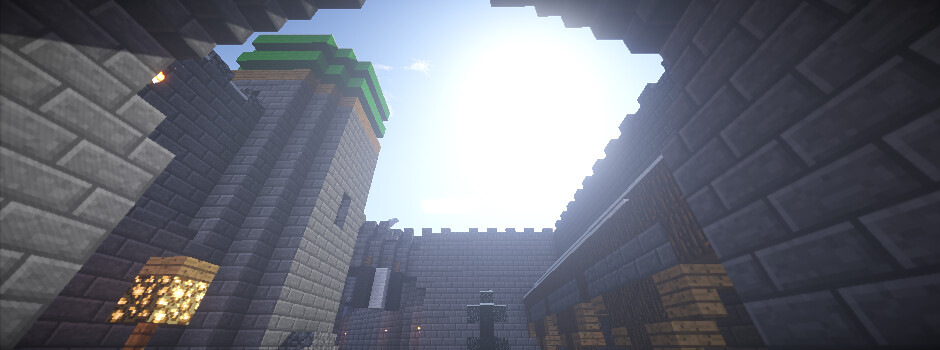This still from a video game depicts a castle courtyard surrounded by imposing gray stone walls, characterized by a scalloped parapet typical of medieval fortifications. On either side of the image, these fortified walls stretch upwards towards a vivid blue sky, partially obscured by the glowing, radiant sun. On the left side, a distinctive tower rises, adorned with two green bands near the top, followed by a brown layer, before culminating in the same gray stonework as the walls below. In the courtyard below, an ambiguous wooden object lies leaned against the stone structure, adding an element of mystery. The scene suggests a game where the player navigates through and explores vast castle environments.